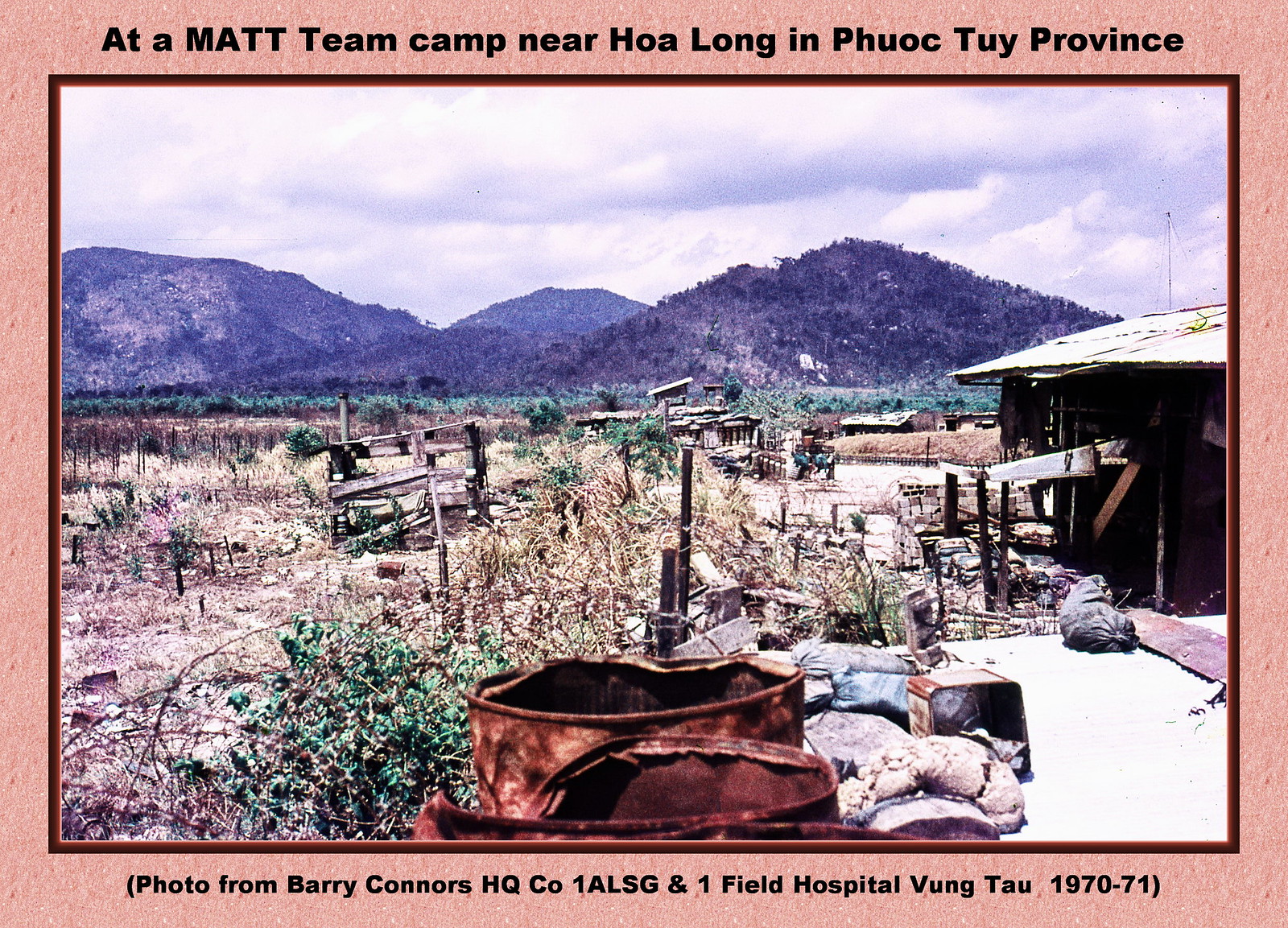This image, reminiscent of a vintage postcard, features a photograph surrounded by a light brown border with an inner pink-red frame. At the top of the border, in black text, it reads: "At a MATT team camp near Hoa Long in Phuoc Tuy Province." The bottom text states: "Photo from Barry Connors, HQ Co 1ALSG and 1 Field Hospital, Vung Tau, 1970-71."

The central photograph captures a rundown country scene. On the right stands a dilapidated wooden shack with a partially metal roof, which appears white, possibly due to sun reflection. The foreground reveals a terrain dotted with old, decaying wooden structures, rusted burn barrels, and torn-down brown fence posts. Scattered around the barrels are dirty white sacks and one large black sack.

To the left of the image is a barren field with dead shrubs, though a few show patches of green. In the distance, three to four brown-hued mountain tops rise against a cloudy sky, emphasizing the desolate ambiance of the camp.